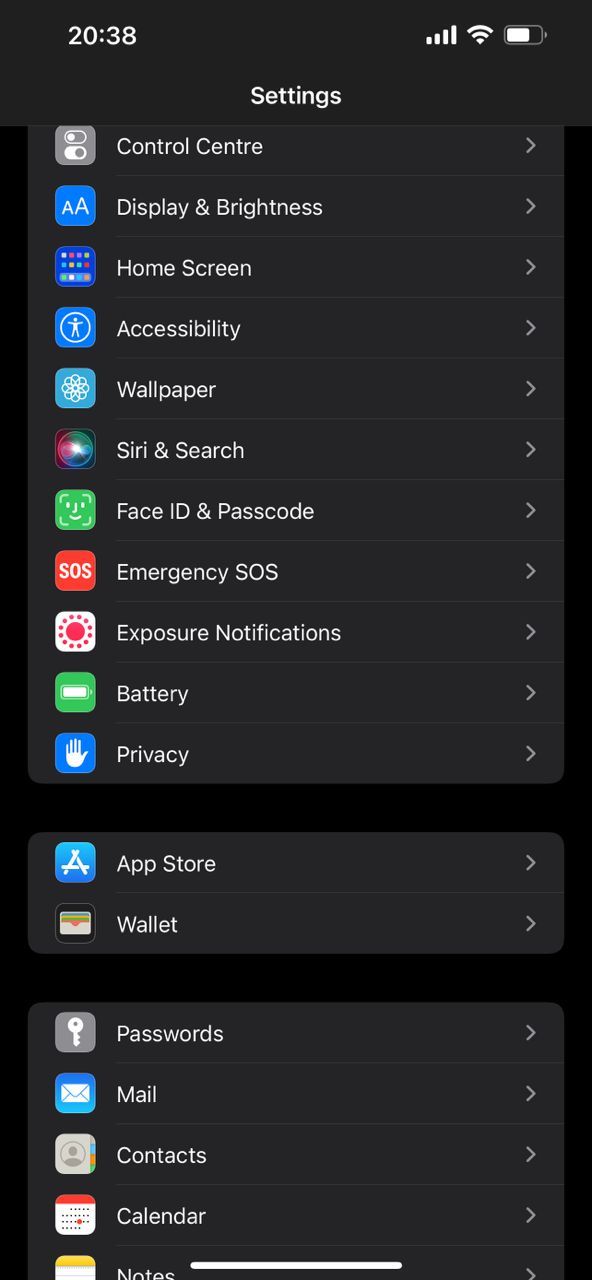The image showcases a smartphone's settings page which features a black background with white text. At the top of the page, the header "Settings" is displayed prominently. A series of settings are listed below, each accompanied by a distinct icon on the left side:

1. **Control Center**: A gray and white icon.
2. **Display & Brightness**: An icon in blue with white "AA" letters.
3. **Home Screen**: A blue icon depicting a home screen.
4. **Accessibility**: A white and blue icon representing accessibility features.
5. **Wallpaper**: An icon in light blue and white.
6. **Siri & Search**: Multi-colored icon with shades of purple, blue, green, and dark hues.
7. **Face ID & Passcode**: A green icon featuring a face scan outline.
8. **Emergency SOS**: A red icon with white "SOS" text.
9. **Exposure Notifications**: An icon in white with red circles.
10. **Battery**: Green icon showcasing a white battery symbol.
11. **Privacy**: A blue icon with a white hand or palm.
12. **App Store**: Blue icon with a white "A".
13. **Wallet**: An icon of a white wallet with green, orange, and blue accents.
14. **Passwords**: Gray icon featuring a key.
15. **Mail**: A blue icon with a white envelope.
16. **Contacts**: A gray icon with a contact log.
17. **Calendar**: White and red icon depicting a calendar layout.
18. **Notes**: White icon featuring a notepad.

Each setting is neatly aligned with its respective icon, making navigation straightforward and visually organized.